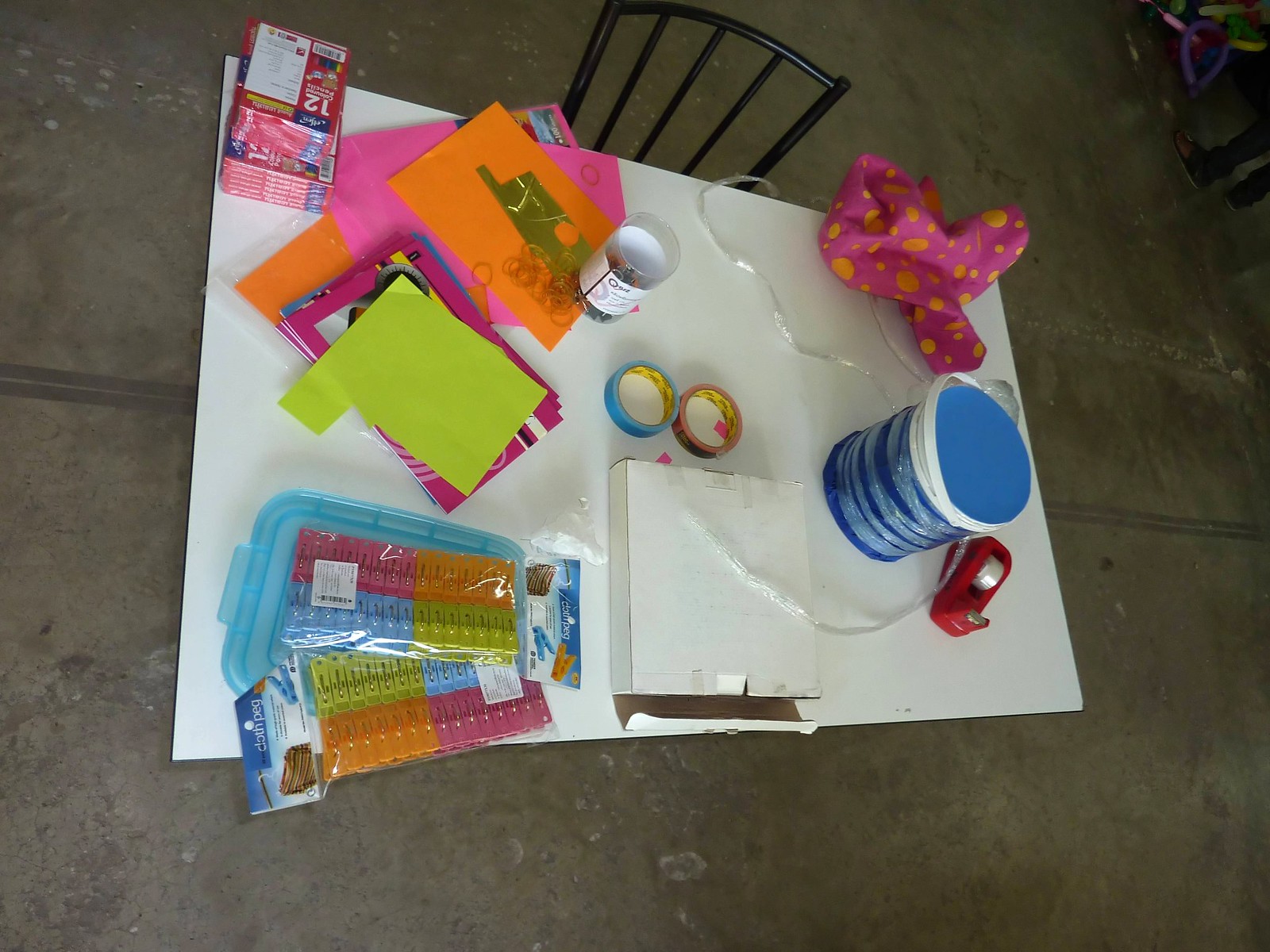The image depicts Anson's workspace. The table, constructed from square tiles resembling cement in brownish hues with some dark gray tones, serves as the focal point. Seated at the table is a black chair, featuring black metal bars on its backrest. Atop the table lies a pristine white poster board, described as "Ming white," surrounded by various arts and crafts supplies.

Scattered across the poster board are vibrant tapes in clear, blue, and neon pink colors alongside various hues of construction paper, including neurofluorescent pink, orange, green, and blue sheets. In the corner of the table is a conspicuous pink hat with orange accents.

Occupying the top corner of the table is a blue plastic container, filled with miniature clips that resemble classic clothespins. These clips are sorted by color—pink, orange, blue, and green—seven clips per color, all packaged together and possibly brand new.

Additionally, a white square box housing rubber bands and a tall, round blue bucket wrapped in clear plastic are also visible on the table, further illustrating the organized chaos of a well-equipped arts and crafts station.